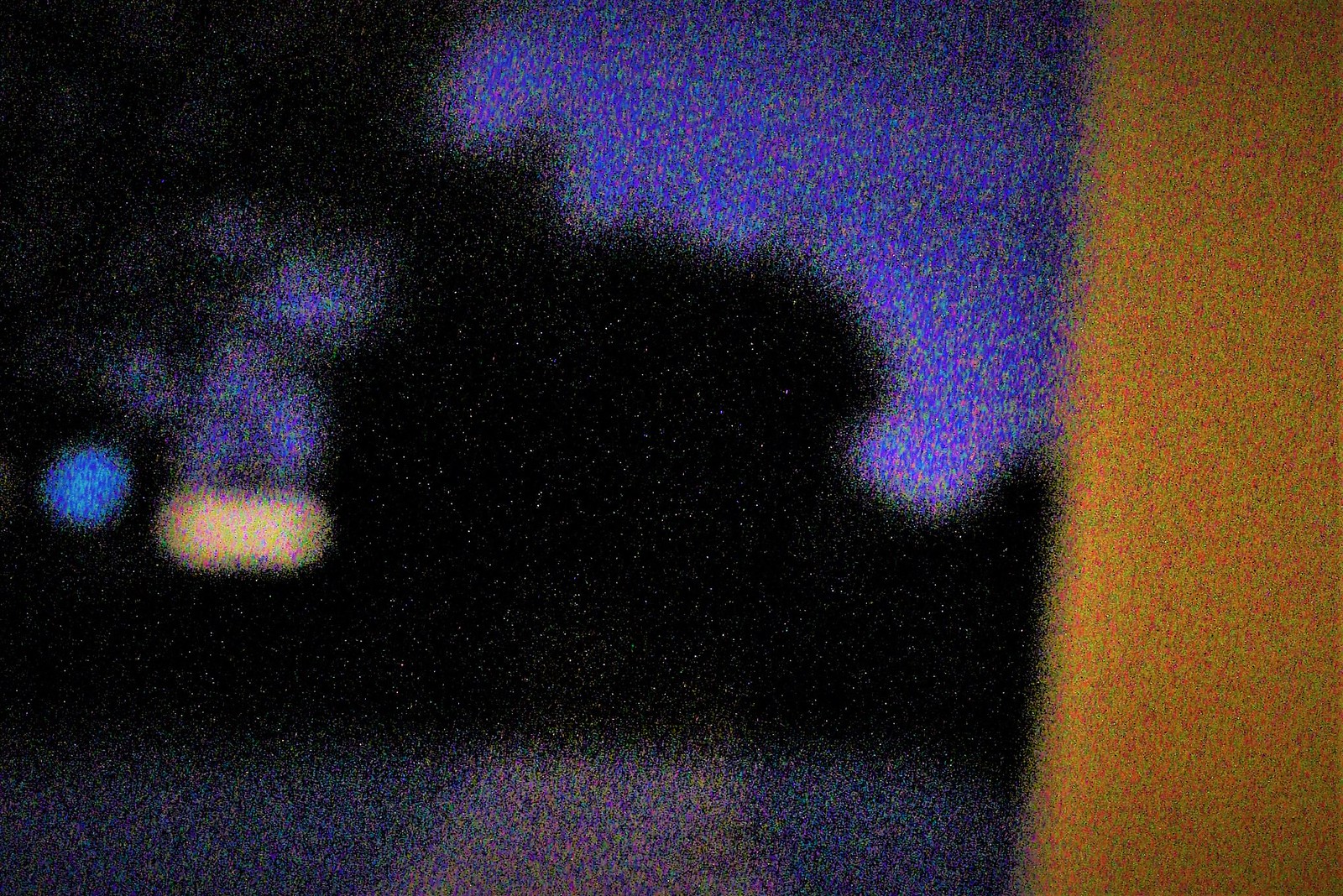This is an extremely grainy and low-quality image that appears to be captured in very dark conditions, making it quite difficult to clearly identify specific objects. The background is predominantly black, resembling a night sky dotted with numerous small bright spots that could be interpreted as stars, suggesting a potential outer space image or an artistic rendering of a starry night. A large, colorful square shape dominates the top central region, with a significant amount of orange to its right. Scattered throughout the image are various colors and shapes: a small, blue circle reminiscent of Earth, albeit inaccurately colored; a yellow, vertical, tapered rectangle in the foreground to the right; and a mix of light purple, blue, and gray hues. In the foreground, at the bottom, there's a grayish circular area with a yellowish line through the middle, adding to the chaos of the composition. To the left, there is a light vertical, football-shaped object, and nearby lies a grainy, bluish blob spotted with white and purple. The overwhelming graininess and distortion suggest the image may have been taken with incorrect camera settings, resulting in a scene that is an ambiguous blend of abstract shapes and colors.